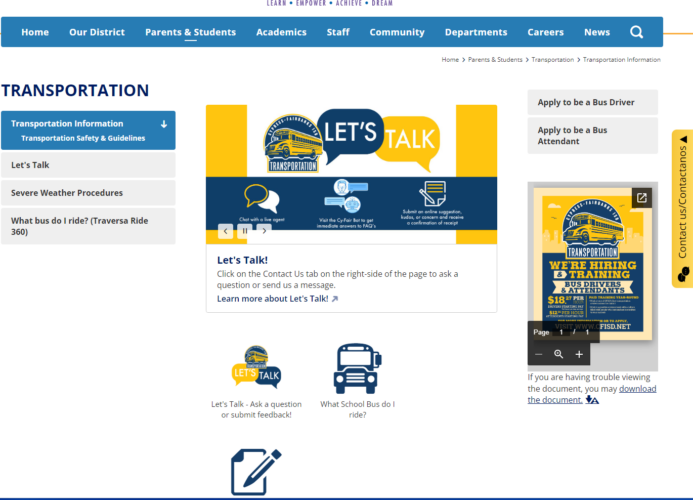The website is designed for individuals interested in applying to be trained as school bus drivers. At the top, there's a prominent blue banner stretching across the entire page with white text indicating different sections: Home, Our District, Parents and Students, Academics, Staff, Community, Departments, Careers, News, and a search icon.

Currently, the viewer is navigating through: Home > Parents and Students > Transportation > Transportation Information.

On the left sidebar, the word "TRANSPORTATION" is displayed in bold blue capital letters. Beneath this header, several subsections are listed, including:

- Transportation Information
- Transportation and Safety Guidelines
- Let's Talk
- Severe Weather Procedures
- What Bus Do I Ride?
- Traversa Ride 360

In the center of the page, there is a feature titled "Let's Talk" with an image of a yellow school bus labeled "Transportation." Below the bus image, there is an invitation to click the "Contact Us" tab on the right side of the page to ask questions or send a message, along with a prompt to learn more about the "Let's Talk" program.

On the right side, two application options are prominently displayed:
- Apply to be a Bus Driver
- Apply to be a Bus Attendant
  
Additionally, there's a small advertisement featuring a school bus icon, which states, "We're Hiring and Training Bus Drivers and Attendants - $18 per hour." Just below, there's a section for contacting in Spanish marked "Contact Us/Contenido en Español." 

An important note indicates that if there are issues viewing the document, users can download it for easier access.

At the bottom of the page, two key options are available: "Let's Talk," where users can ask questions or submit feedback, and "What School Bus Do I Ride?"